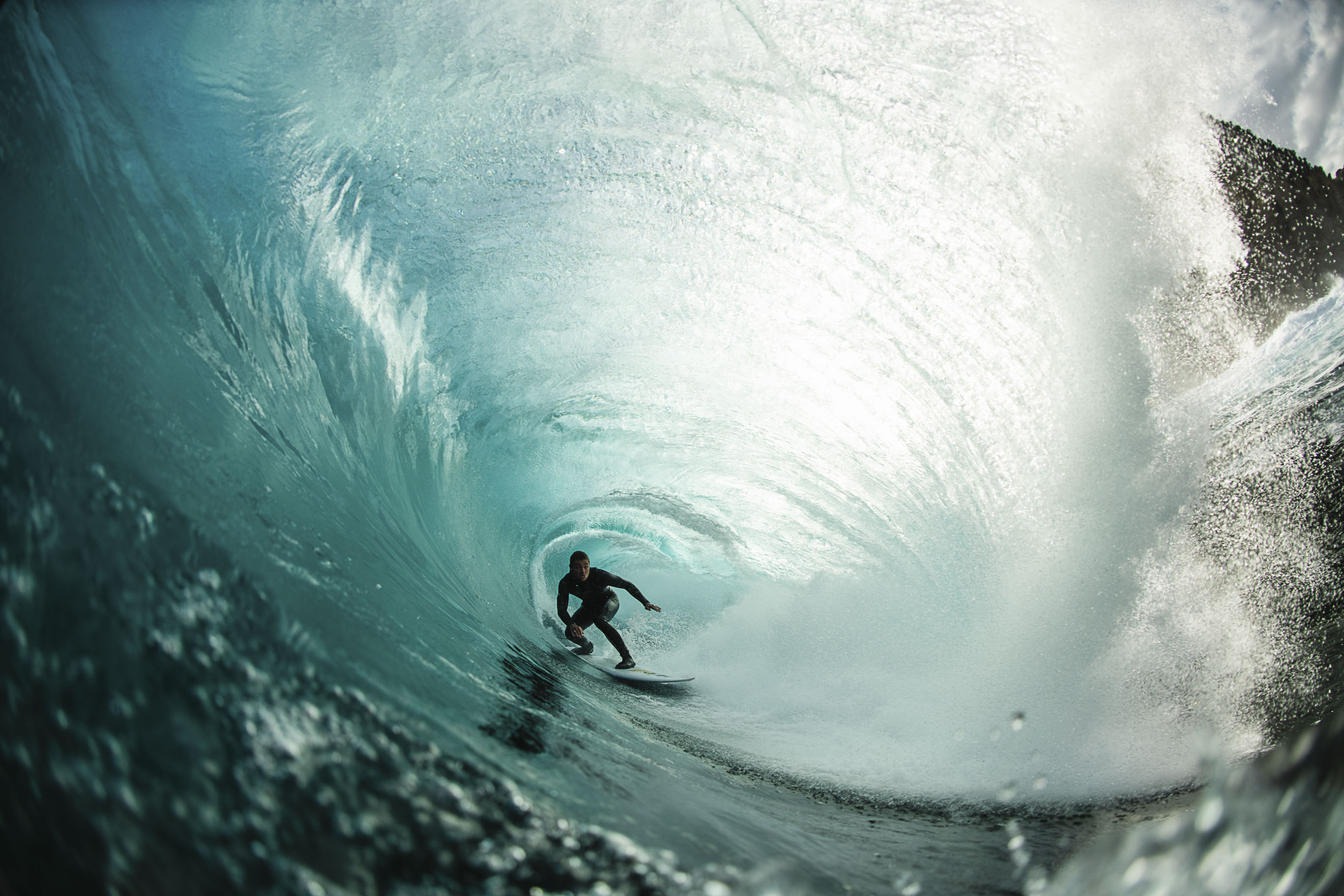This landscape photograph captures an exhilarating moment of a surfer performing a "hang ten" maneuver inside a tubular wave. Viewed from the side and slightly in front as if from another surfer's perspective, the image immerses us in the dynamic scene. The horizon line curves dramatically due to the warped lens effect, with the right side of the image showcasing a rugged shore and rocky hills under a cloudy sky. The wave itself cascades elegantly over the surfer, exhibiting a mesmerizing gradient of dark aqua, blackish-blue, and glassy light blue hues, punctuated by white spray.

At the heart of the image, the surfer, adorned in an all-black wetsuit that includes a hood, rides a light blue surfboard while crouched in a focused stance. Their left arm extends outward, their right arm tucks beneath them, and both knees are bent, embodying the fluidity and control required for such a daring ride. The wave's powerful curvature creates a captivating vortex, almost tunnel-like, through which the surfer glides. The translucent, almost white water behind the surfer, illuminated by the sun, contrasts sharply with the darker tones around, adding to the image's dramatic intensity. The overall scene is a harmonious blend of motion, color, and light, encapsulating the thrill and beauty of surfing within a perfectly timed and visually striking moment.